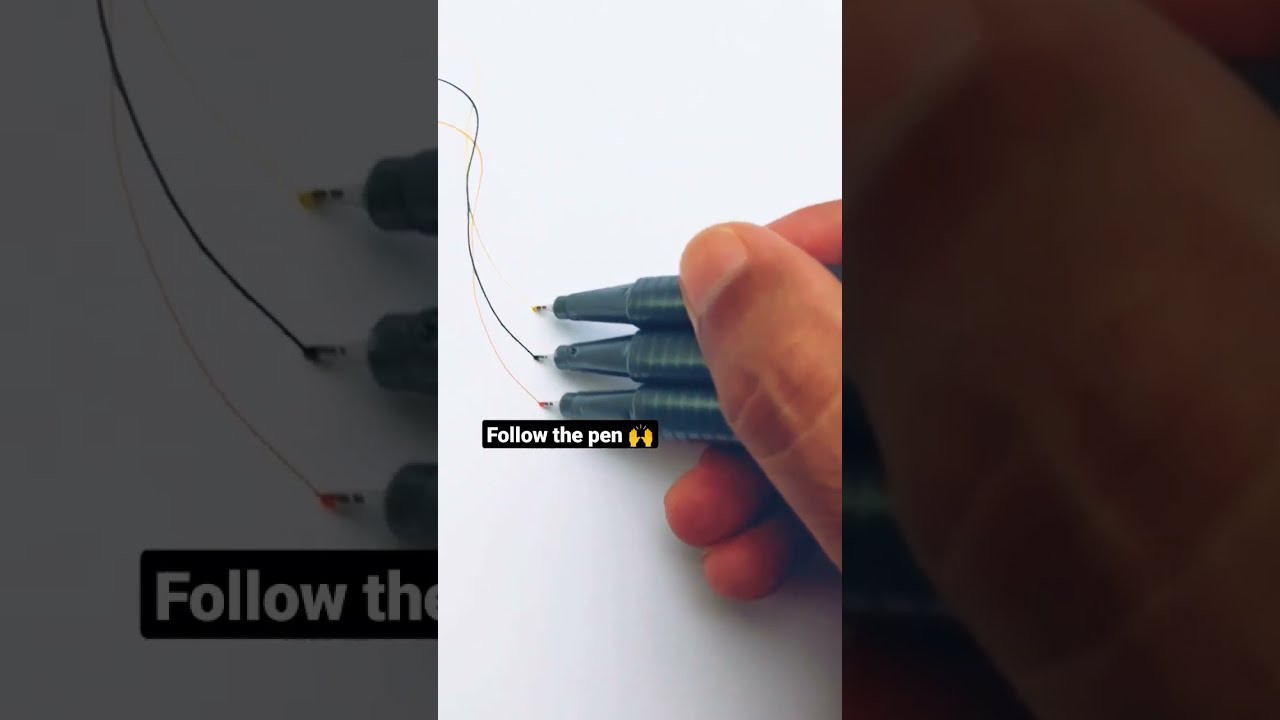The image captures a close-up of a right hand holding three pens, each with a different ink color—yellow at the top, blue in the middle, and red at the bottom. The pens are held between the thumb and index fingers, actively drawing a curving line on a white piece of paper. This line crisscrosses and varies in intensity based on the pressure applied. Above the pens, there's an Instagram overlay with the text "follow the pen" in white font on a small black background, accompanied by a hands-up emoji. The entire scene is layered over a darkened, blown-up version of the same image, which serves as the background, emphasizing the details of the drawing and the hand's movement. The person's fingers appear neatly clipped as they drag the pens along the paper.